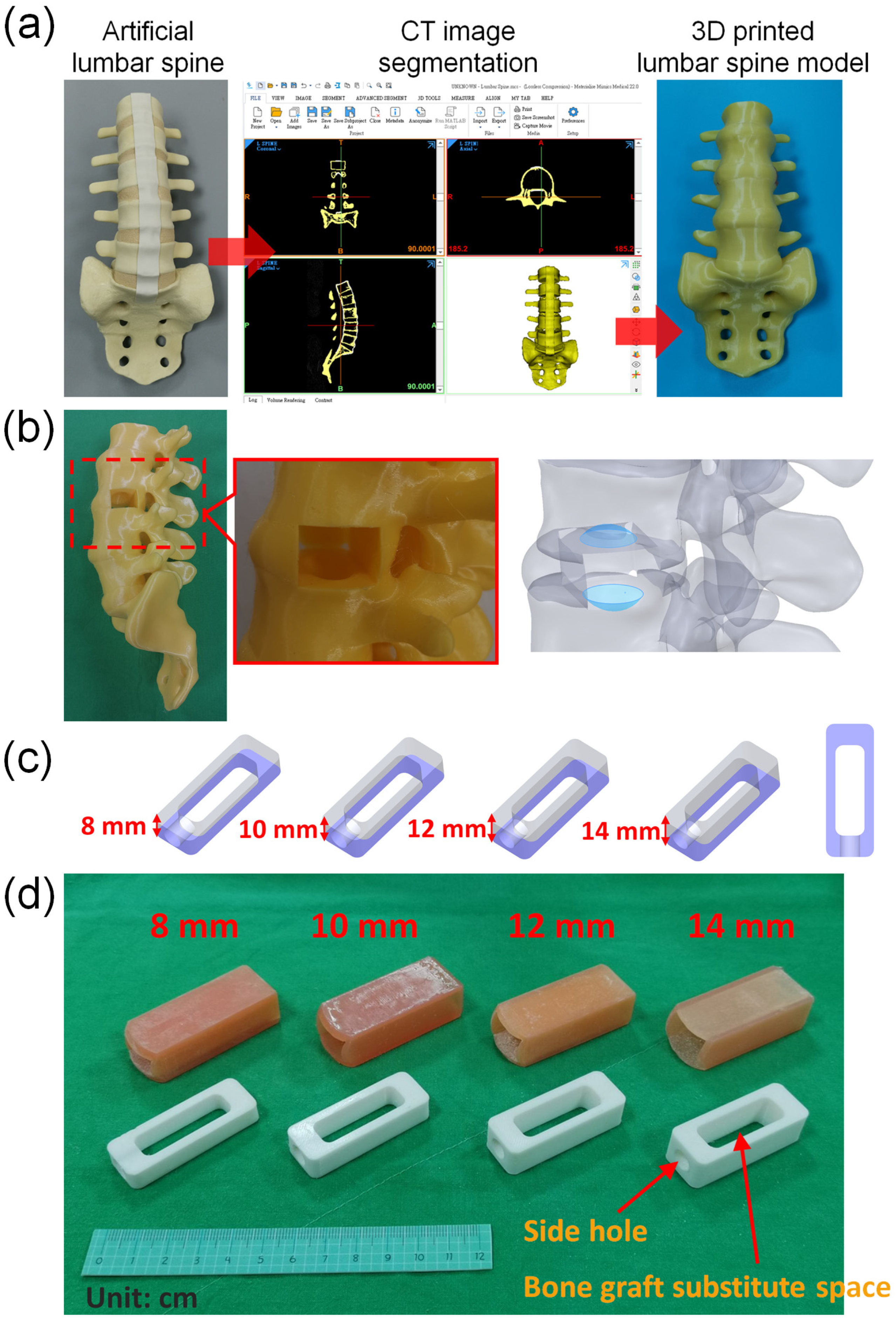This vertically aligned rectangular image, devoid of any border, serves as a detailed illustrative flyer seemingly focused on advancements in medical technology, specifically related to the lumbar spine. The image is meticulously labeled with lowercase alphabet letters (a-d) on the left side, arranged from top to bottom in black text.

In the top-left corner (labeled 'A'), there is a title "artificial lumbar spine," accompanied by an image of a white artificial lumbar spine. To the immediate right, a red arrow points towards the sub-caption "CT image segmentation," which is depicted through a series of four small images displayed on a computer screen. On the upper-right portion of the image, the title "3D printed lumbar spine model" is presented alongside an illustrative representation of such a model.

Beneath this section (marked 'B'), there are three images, but these are not described with any accompanying text. Proceeding further down to section 'C', the image displays a series of small rectangular purple and gray figures, each indicating different depths - specifically 8mm, 10mm, 12mm, and 14mm - with these measurements highlighted in red print. Finally, the bottom section ('D') presents a large green rectangle showcasing various graphs related to "bone graft substitute space," with all measurements provided in centimeters. Additionally, there is a ruler laid out within this section, further emphasizing the precision of the measurements.

Overall, this image documents and illustrates multiple facets of spinal medical advancements, including artificial lumbar spines, CT image segmentation, and 3D printed lumbar spine models, structured in a clear and sectioned manner.